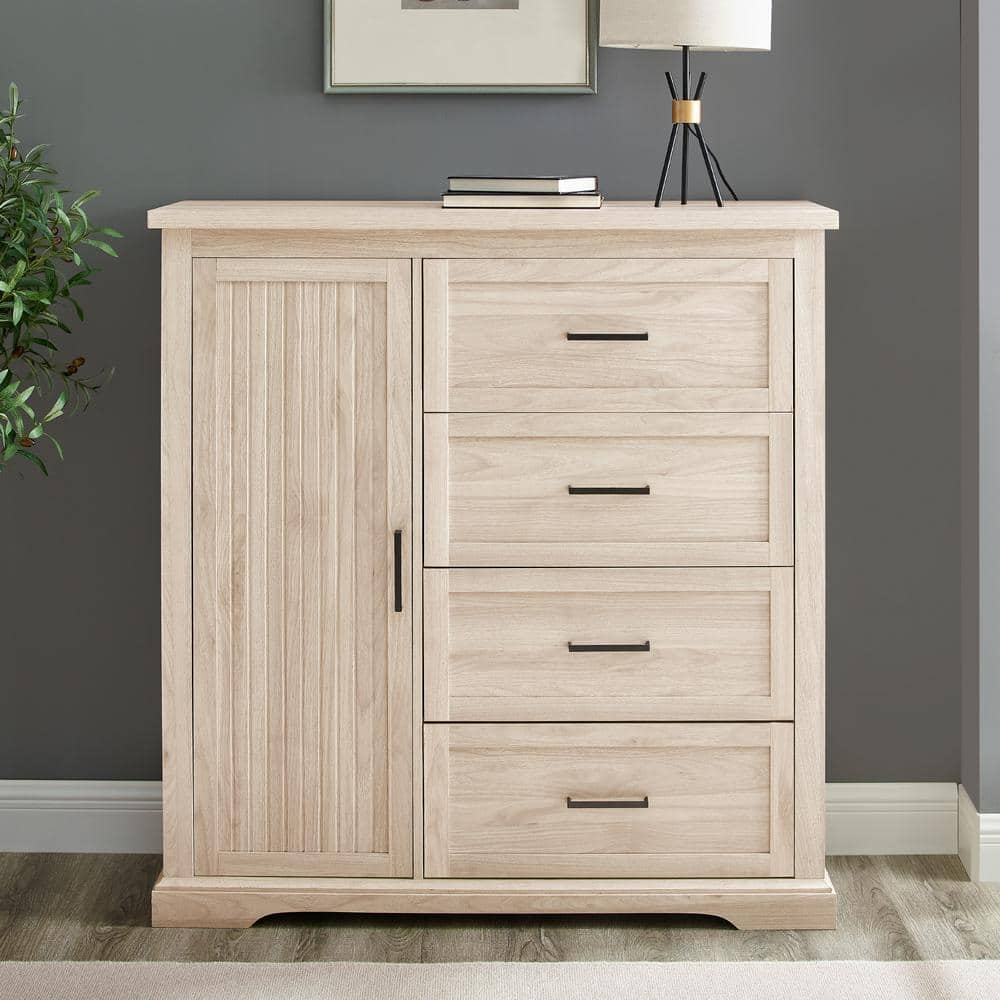The photograph captures an indoor setting featuring a modern, light brown wood dresser with a sleek, minimalistic design. The dresser has a vertical cabinet door on the left side, equipped with a metal handle, and four horizontally-aligned drawers with black handles on the right. It stands against a grayish-blue wall that complements the brown wooden floor below. On top of the dresser, there are two hardcover books with their spines facing the wall, and a modern black lamp with a white lampshade, featuring a tripod-like support with a visible power cord. Above the dresser, slightly to the left, hangs an off-frame painting. Additionally, green leaves from a plant or small tree partially enter the frame from the left side. The room also has a white rug covering part of the wooden floor at the bottom of the photograph, and a hint of natural light suggests the presence of a window off-frame to the right.